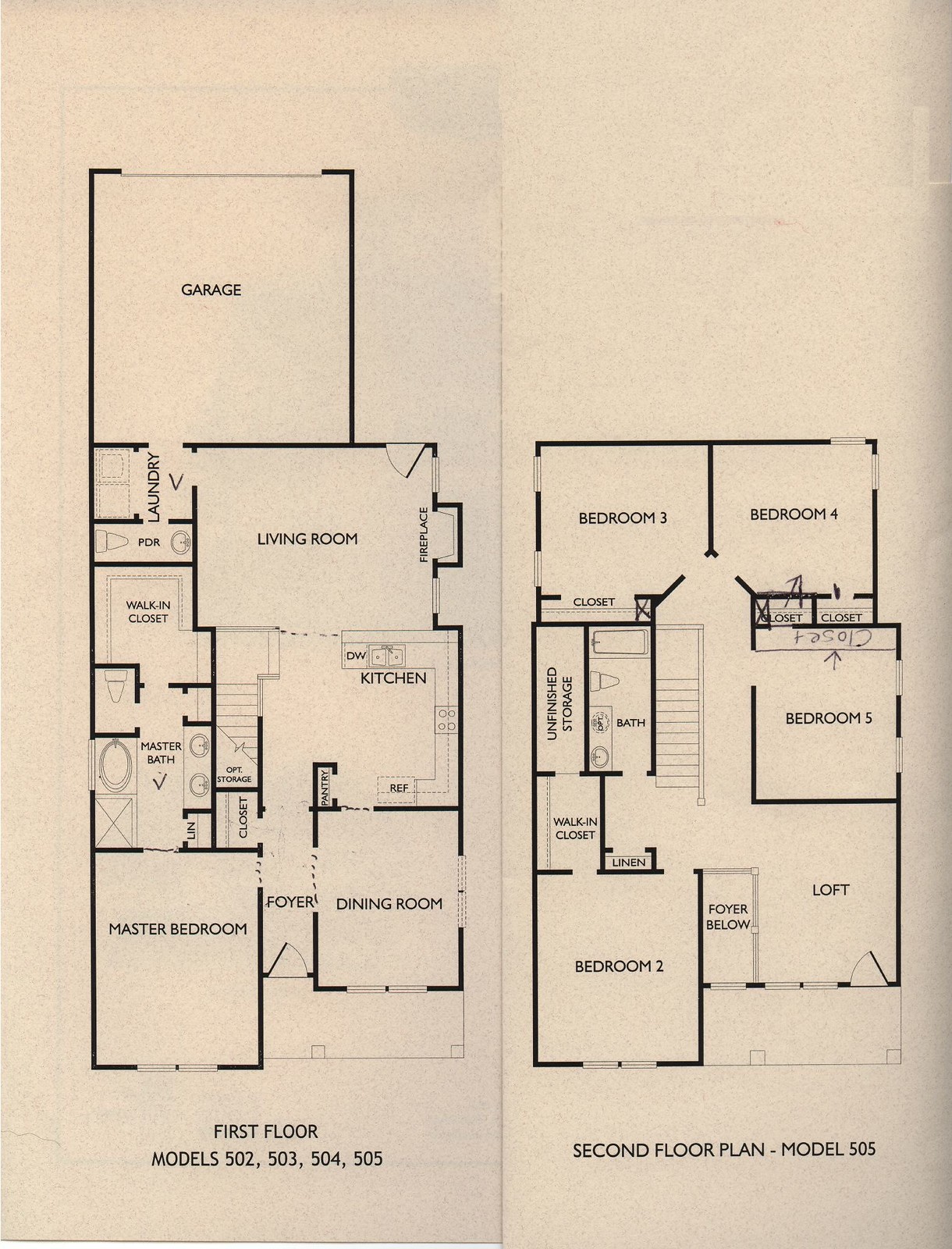The image appears to be a detailed floor plan of a house with clearly labeled rooms for both the first and second floors.

**First Floor:**
- The left side of the image is oriented vertically. At the top left, a black box labeled "Garage" is prominent.
- Adjacent to the Garage is a smaller square labeled "Living Room" and further left, an even smaller square marked "Laundry" with an arrow pointing downwards.
- Directly below the Laundry, connected by an arrow, is a square labeled "Walk-in Closet."
- Continuing downwards with another arrow, the next square is marked "Master Bath."
- At the bottom of this vertical sequence is a larger square labeled "Master Bedroom."
- To the right of the Master Bath is the "Foyer," and further right, a larger box labeled "Dining Room."
- Above the Dining Room is a designated "Kitchen" area, which also shows outlines of kitchen counters.
- Finally, the square located above the Kitchen is labeled "Living Room."
- Along the bottom of the image, the text reads "First Floor Models 502, 503, 504, and 505."

**Second Floor:**
- The second image on the right is smaller and starts with two adjacent squares at the top: "Bedroom 3" on the left and "Bedroom 4" on the right.
- Below Bedroom 4 is another square marked "Bedroom 5."
- Adjacent to Bedroom 5 is a square labeled "Loft."
- To the left of the Loft is the "Foyer," situated below.
- To the left of the Foyer is a black square labeled "Bedroom 2."
- Moving upward, connected by arrows, is "Walk-in Closet," and above that, to the right, the "Bath."
- Above the Bath, another compartment is labeled "Closet," and to its right is "Bedroom 1."
- At the bottom, small text reads "Second Floor Plan - Model 505."

This organized description provides a clear and detailed overview of the house's layout and room types across both floors.